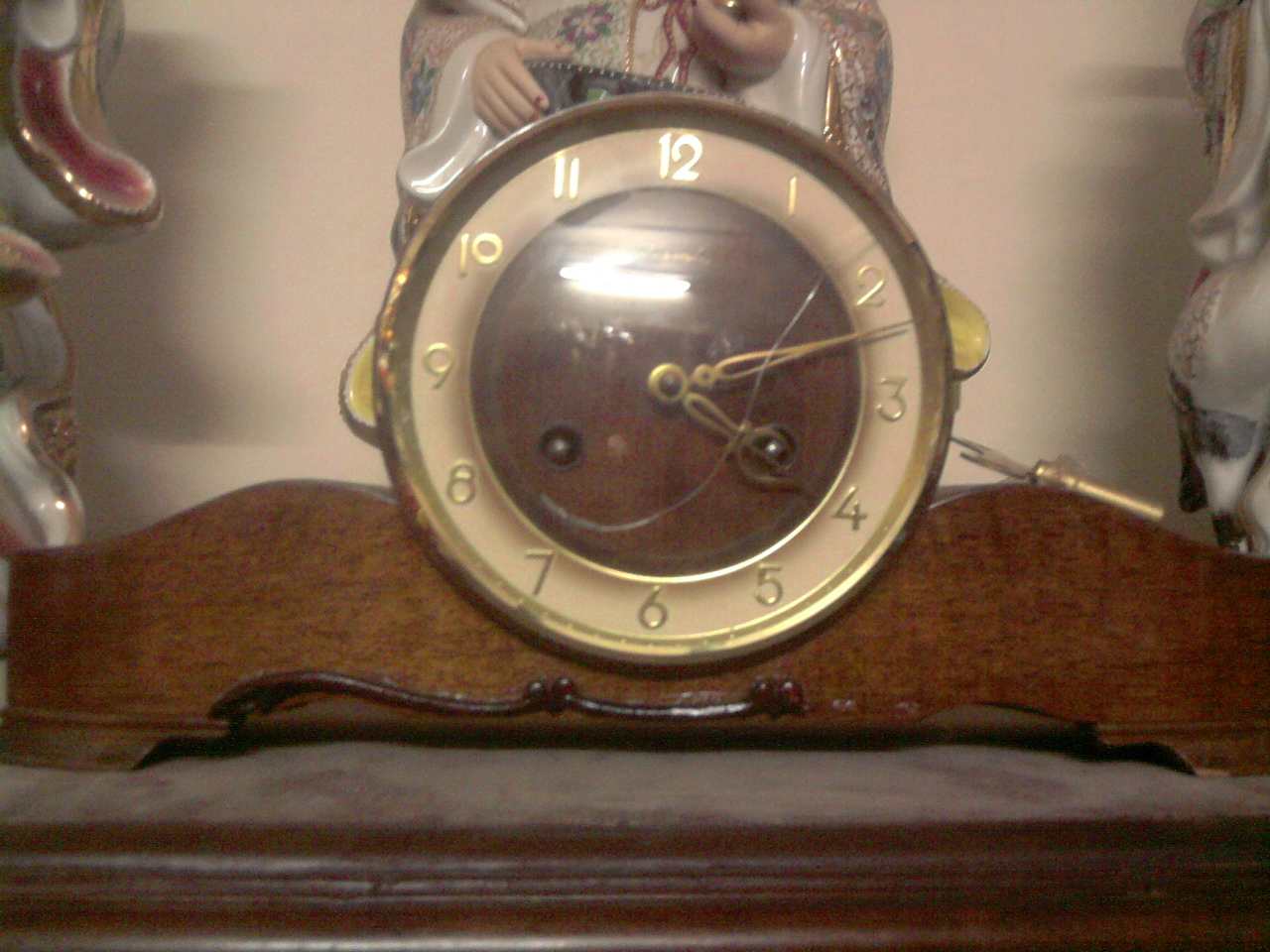The image showcases an antique clock with a distinctive, ornate design. The clock features a brown rim and center with a golden ivory face, where the golden numbers and hands elegantly indicate the time, reading approximately 4:12. The clock rests on an intricately crafted wooden stand, adorned with elaborate dark wood scrollwork and a noticeable layer of dust. Perched atop the clock is an elegant sculpture of a woman, while a horse figurine stands to the right. The background reveals a collection of beautifully crafted ceramic figurines, including one wearing a tan robe with blue flowers. The scene is set against a tannish white wall with a shadow crossing through the center, adding to the antique charm of the display. The setting suggests the clock and surrounding objects are cherished pieces, adding to the overall historical and artistic value of the scene.